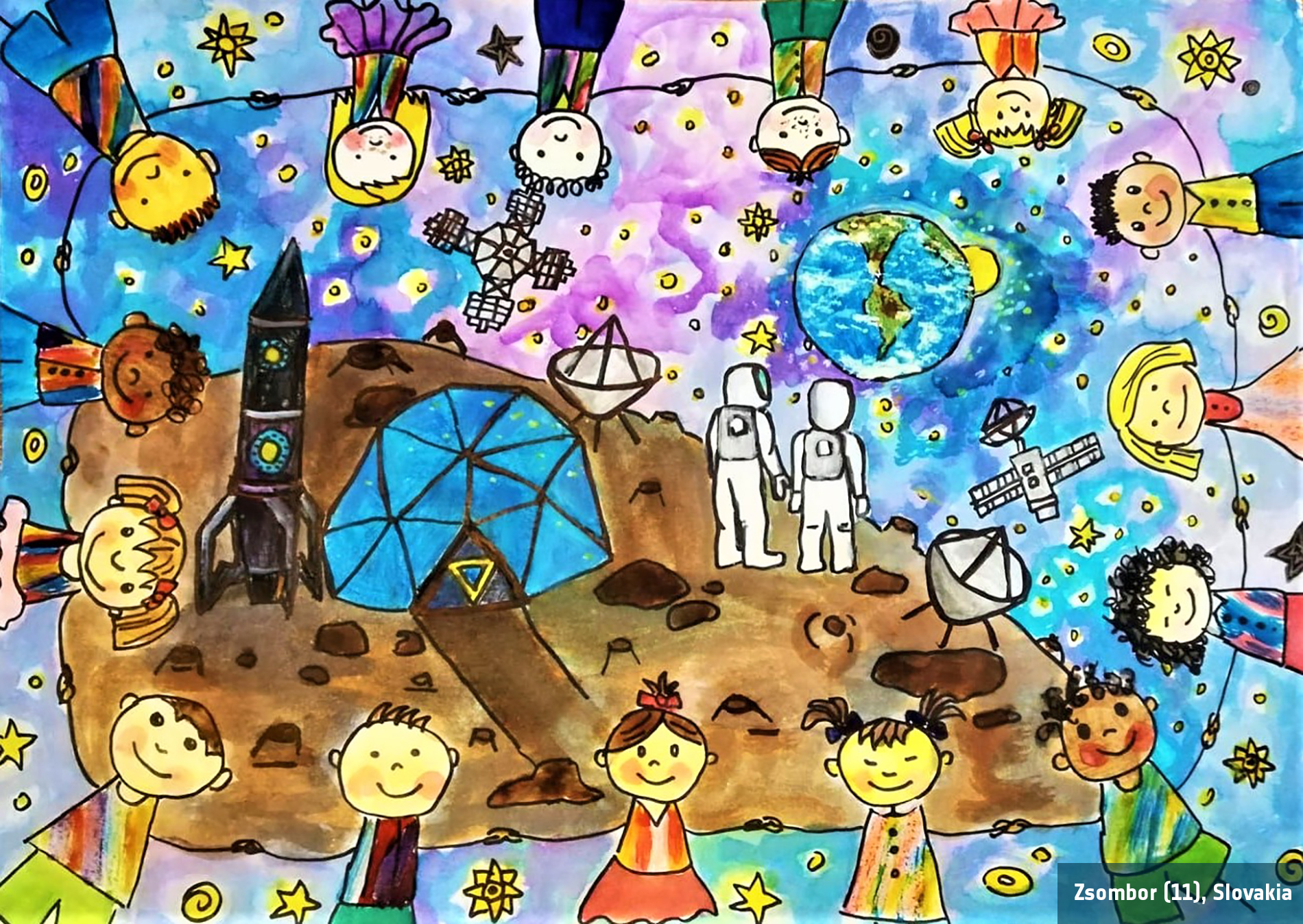The image resembles a child's vibrant watercolor drawing, featuring a captivating blend of purples, blues, and pinks to depict a night sky, sprinkled with various star shapes. Surrounding this celestial scene, children of diverse races and genders are drawn in a chain, holding hands along the borders of the image—some upside down, sideways, or right side up, making a continuous, cheerful loop around the rectangular frame.

At the center of the picture, the artwork portrays what appears to be a moon landing. The brown, uneven lunar surface with small craters is home to two astronauts in white suits, their visors tinted greenish-blue, gazing contemplatively at the distant Earth. Nearby, there stands a black rocket ship and a blue, dome-like structure resembling a tent, composed of triangles with a distinctive pattern of a brownish base, a yellow downward-pointing triangle, and a blue triangle within it. This scene also includes two white satellite dishes—one to the left of the structure and one to the right—along with additional satellites equipped with solar panels floating in space.

Finally, in the bottom right corner of the drawing, the text "ZSOMBOR (11), Slovakia" is inscribed in white font, adding a personal touch to this imaginative and richly detailed depiction.